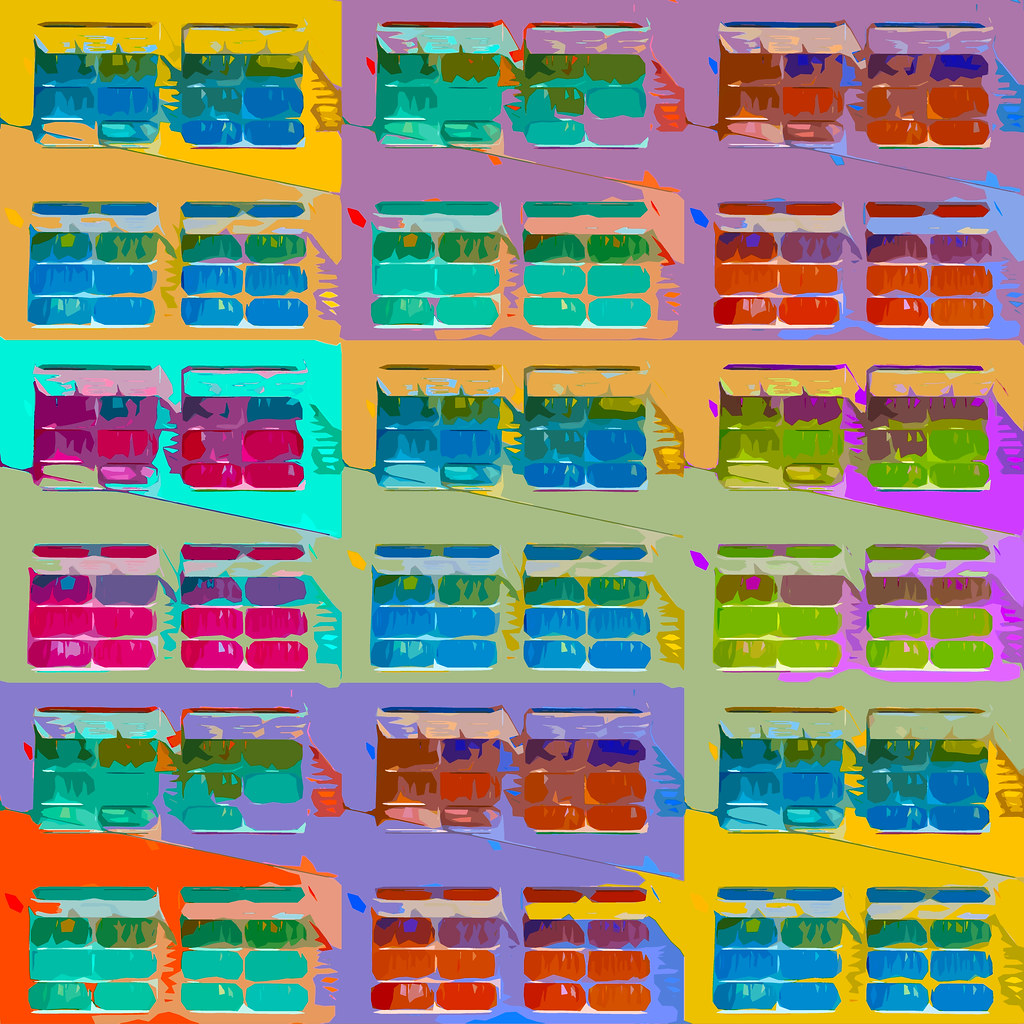The image is an extremely colorful piece of pop art reminiscent of Andy Warhol's work. It features nine rectangular sections arranged in a grid, each depicting a repetitive pattern that resembles factory or garage windows with small overhangs. Each rectangle showcases vibrant and varied color schemes, using combinations of yellow, blue, purple, green, red, turquoise, sage, mint, electric green, and electric orange. The image appears busy and dynamic, inviting viewers to explore its multiple hues and designs. Some rectangles include a distressed effect with additional colors layered into the primary ones. The sections are separated by line elements, which might resemble mascara or eyeshadow palettes in shades of purple, blue, green, and red, adding to the intricate and engaging composition.